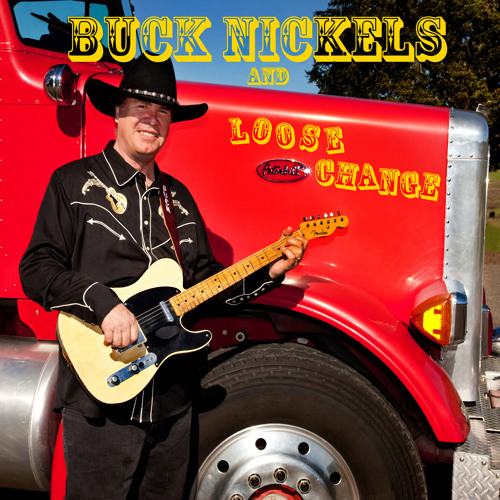The photograph depicts a Caucasian man in a country-western outfit, possibly for a musician's CD cover or bar advertisement. He is standing outdoors in front of a red Peterbilt semi-truck, easily recognizable by its logo. The man, identified as likely being part of the band "Buck Nichols and Loose Change," is dressed in black jeans, a black button-down shirt with white and reddish trims and an embroidered guitar, and a black cowboy hat. He holds a distinctive yellow and black electric guitar, fingering a chord on its neck with his left hand. The image features text in yellowish and bluish hues that reads "Buck Nichols and Loose Change," positioned around him. The scene is naturally lit, with visible details of the truck's silver front, large tire, pavement, grass, part of a tree, and the sky in the background. The man gazes directly at the camera, capturing a striking and vibrant portrait.